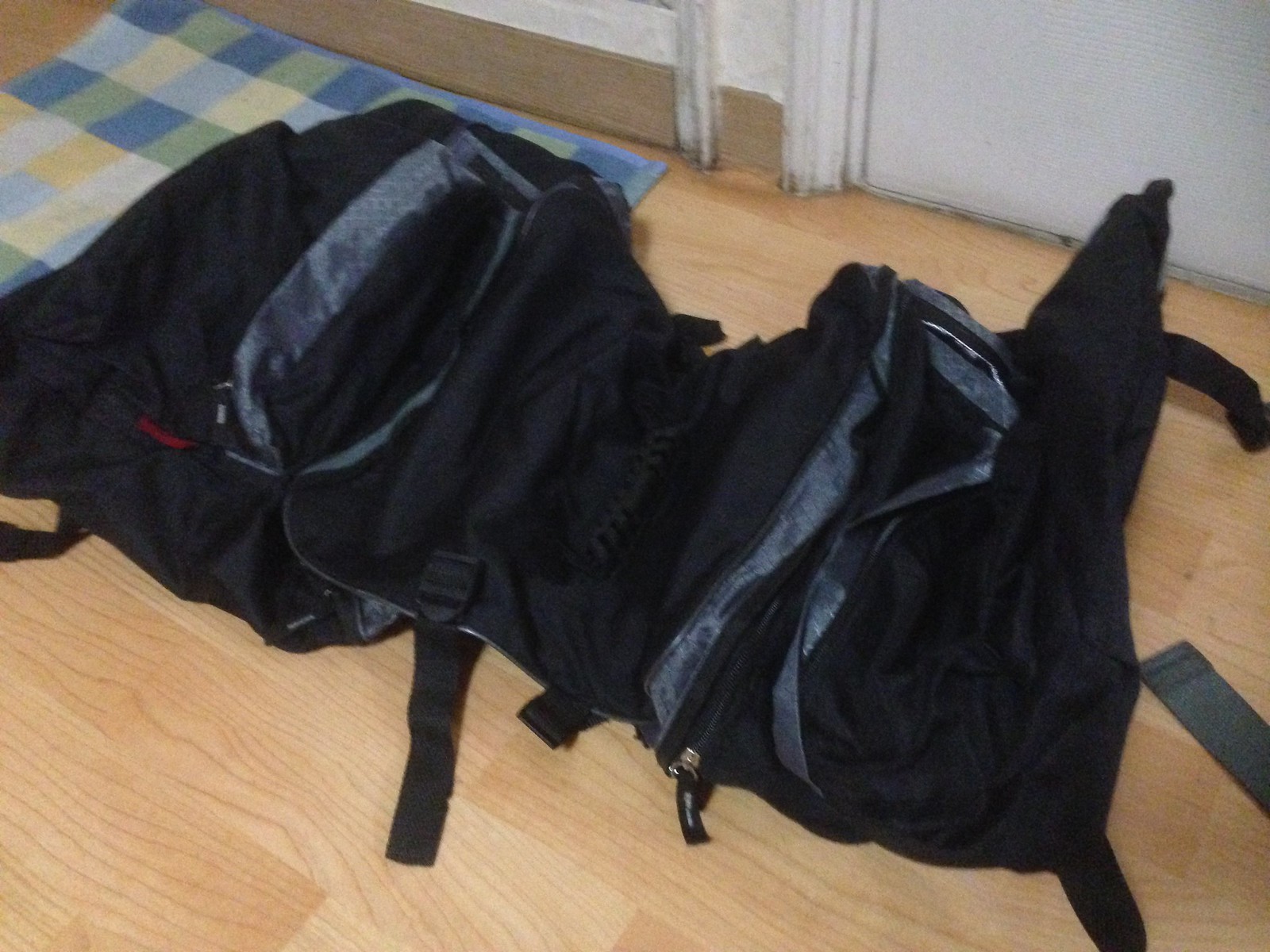In a horizontal rectangular photograph, a black and deep green folding travel bag lies open on a light laminate wood floor. The bag, which can fold into itself, features various wide pockets, zippers, and shoulder straps. The floor, with a synthetic wood grain pattern, extends to the upper right of the image, where part of a dingy off-white door and its tan baseboard trim are visible. Near the door is a multi-patterned blanket or small area rug with shades of blue, yellow, green, and white. The area rug has blue binding around the edges. The focus of the photograph is somewhat blurry, adding to the overall casual and lived-in atmosphere of the scene.